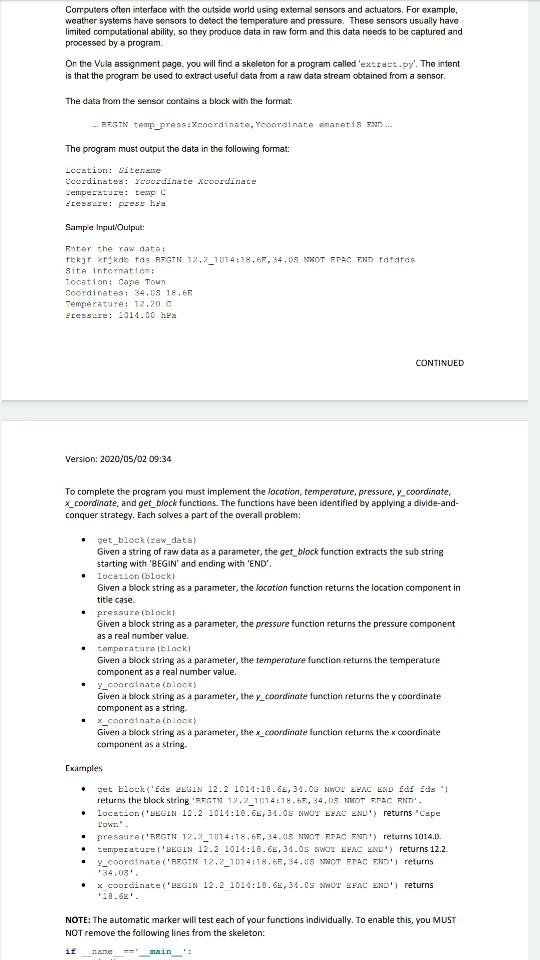This image shows a screenshot featuring two pages from a user manual or programming documentation. The pages are predominantly white, and there is a visible overlap with the bottom of the top page displaying the word "continued." The text on these pages is minimal and difficult to read at the current scale of the image.

The top of the first page begins with a paragraph in bold black text, followed by code segments integrated within subsequent bold text headings. Further down, an indented line of programming code appears beneath another bold text section, accompanied by more descriptive black text followed by four additional lines of code. As the page progresses, there's a section labeled "Sample Input Output" in bold text, with numerous lines of code beneath it. The bottom of this first page concludes with the word "continued."

The second page starts similarly with a paragraph of bold black text followed by a bulleted list. Each bullet point comprises a brief line of programming code accompanied by a line or two of descriptive black text. Toward the bottom of the second page, there's a heading in bold black text labeled "Examples," followed by another bulleted list containing more code or settings details. Overall, these pages provide a structured mix of textual explanations and coding examples typically found in technical manuals or programming guides.